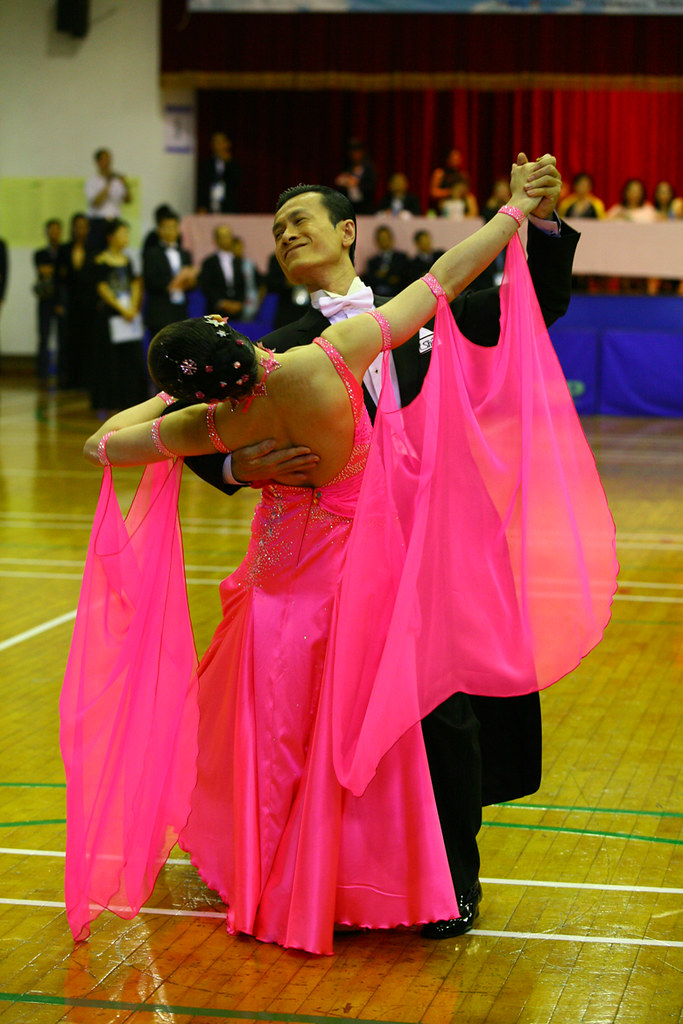The image captures an enchanting moment from a dance tournament. The focal point is a male dancer gracefully supporting a female partner who is striking an elegant pose, bent backwards. She is adorned in a striking, hot pink dress that flows beautifully and features sheer, cape-like arm accessories fastened with three straps on each arm, creating an ethereal "wing" effect when she extends her arms. Her dark hair is elegantly styled in an updo and decorated with pink and white ornaments, complemented by a matching pink necklace. The male dancer is impeccably dressed in a long black tuxedo coat that extends about a foot above his ankles, paired with a white shirt, white bow tie, and black buttons. Behind them, the scene is set in what appears to be a gymnasium with vinyl flooring, where other contestants await their turn in similarly elegant attire. A stage can be seen in the background, likely where the judges are seated, observing the captivating performances. Spectators also line the background, fully immersed in the dance spectacle before them.